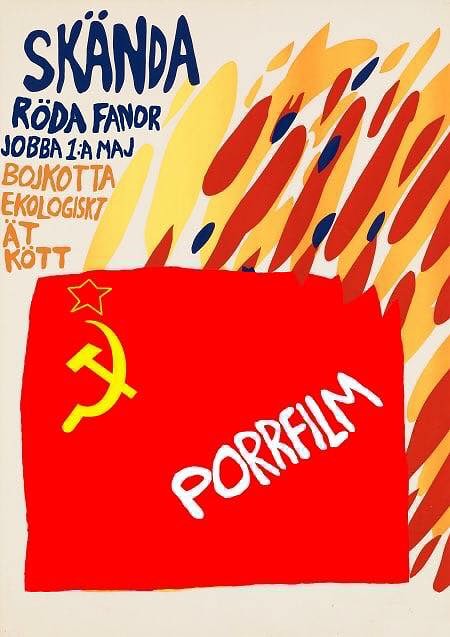The illustration features a light pink background with roughly hand-drawn, irregular shapes and symbols. In the upper left corner, there is text written in capital letters. At the top, it reads "SKÄNDA," with two little dots over the first 'A', followed by "RÖTA FENOR," also with the same marked 'O'. Below this, the text includes "JABBA 1:A MAJ," and "BOJKOTTA" all handwritten in an uneven and painted style with tan-colored font. In the center of the image, there is a large, misshapen red rectangle with a golden hammer and sickle and a star above it, resembling Soviet iconography. Inside this rectangle, the text "PORR FILM" is depicted diagonally in a playful white font. Surrounding and slightly emerging from this red rectangle are colorful blobs and dots in red, yellow, orange, and blue, adding to the hand-painted aesthetic.